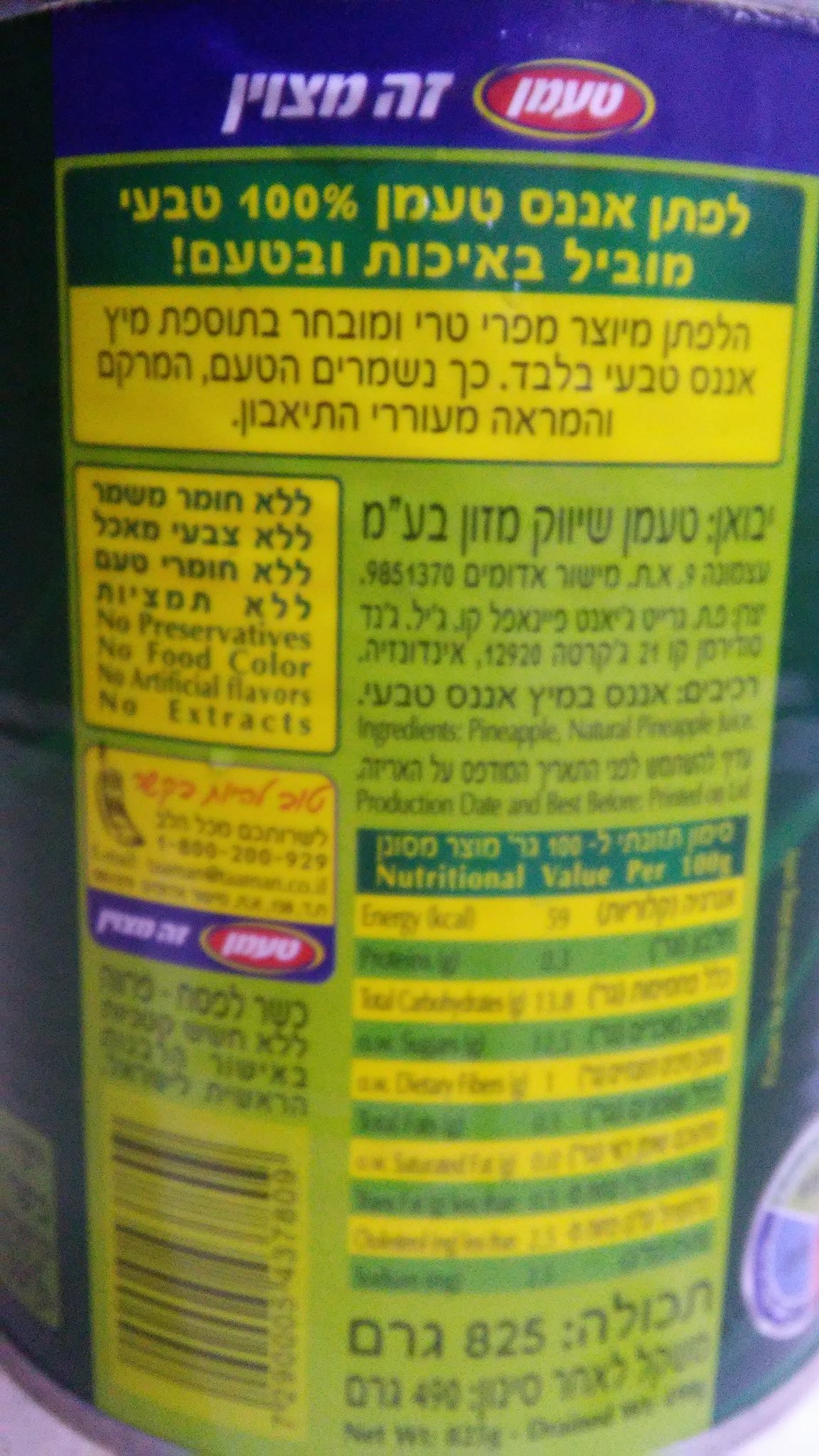The image showcases the backside of a cylindrical canned food container, zoomed in for a close-up view. The label, predominantly dark blue around the edges, features a vibrant and colorful design with squares of purple at the top, transitioning to green, yellow, and lime green sections. These squares contain various nutritional facts and text in a language that is not English, though some parts appear in English detailing the nutritional value per 100 grams: energy 59 Kcals, proteins 0.3, and total carbohydrates 11.8, with 0% sugars. The text layout includes dark green with yellow text, followed by black text on a yellow background, and continues in a pattern of yellow and green squares. There is also a small red oval shape with a yellow line around it near the top. The entire label appears detailed but parts are blurry, especially toward the bottom where the net weight is partly visible but unreadable. The can is sitting on a light-colored flat surface, adding to the overall detail of the image.